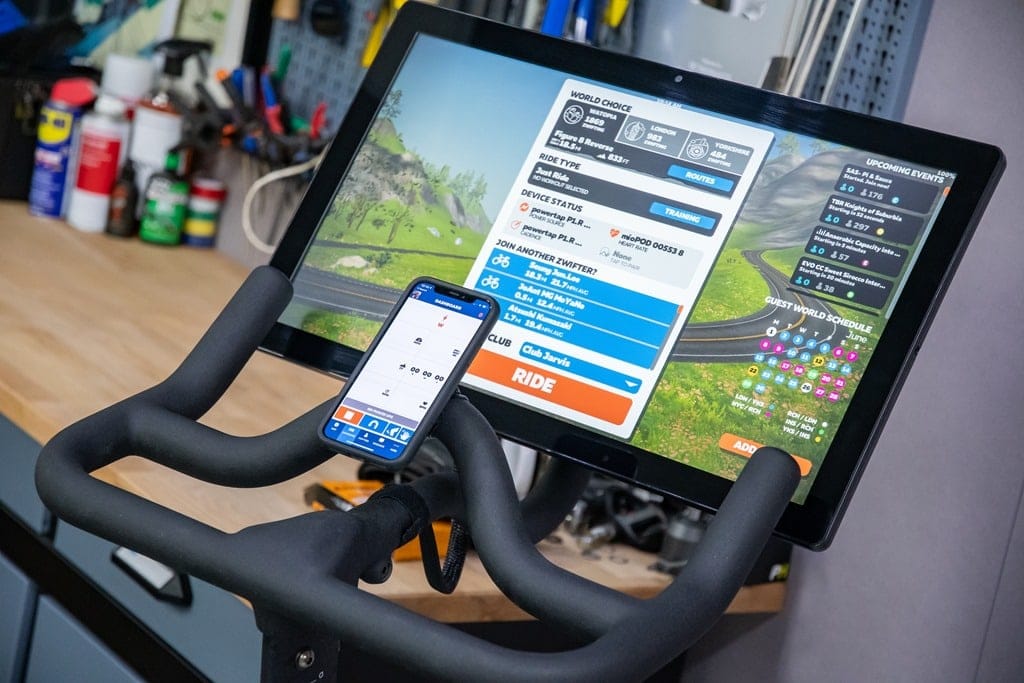The image showcases a close-up of an exercise bike's screen, prominently featuring the handlebars with a mounted smartphone displaying an app. The exercise bike is situated in a garage-like environment, with a workbench visible in the background, cluttered with various tools, WD-40 cans, and other typical garage items. The large rectangular screen on the bike displays a virtual scene of a winding road leading towards mountains surrounded by grassy fields and wildflowers. The screen's interface includes a white page titled "World Choice," featuring gray, blue, and orange accents, with the word "Ride" in orange at the bottom. The interface also presents several interactive options allowing users to join rides with others. The image provides a detailed glimpse into a mix of fitness and function, set against the backdrop of a typical home garage workspace.